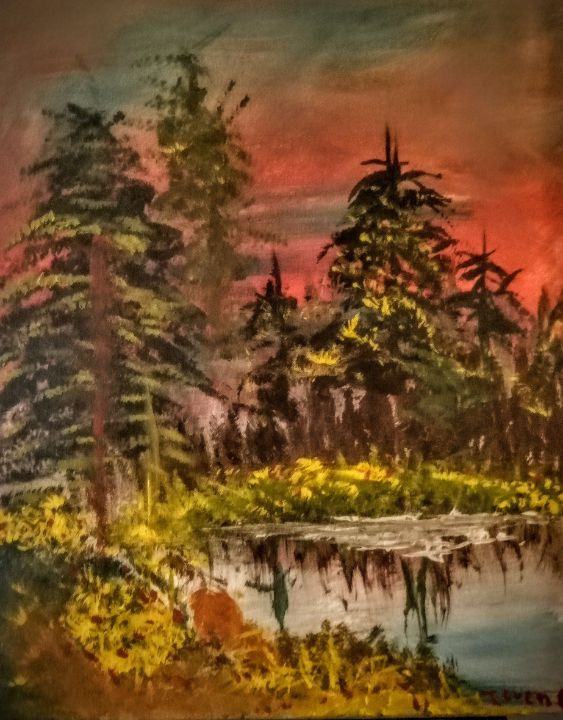This painting is a beautifully detailed oil painting capturing a serene lakeside forest landscape. The artwork is oriented in portrait mode and features a reflective bluish-white lake or pond that extends from the bottom right corner into the lower center of the image, adorned with white foam at the shoreline. Along the shore, dark green plants with light yellow flowers and some reddish blooms emerge, blending into brown patches of earthy grass.

Dominating the mid-ground are tall pine or evergreen trees, reminiscent of Christmas trees with their green leaves and robust brown trunks. Three prominent trees are centered, peeking out behind a backdrop of additional firs and pines that infuse the scene with depth. The foreground greenery is complemented by the reflection of these trees on the water's surface, adding an extra layer of visual interest.

In the lower left corner, a small, somewhat indistinct figure of a woman is slightly bent over, seemingly engaged in an unknown activity. Above this tranquil scene, the sky becomes the focal point with its striking colors—soft, dusky pinks and grays blend with a darker gray as it stretches upwards, hinting at an impending sunset. 

The overall painting style is characterized by broad brown strokes for the tree trunks and textured, horizontal brushstrokes that depict the dense green foliage. The artist’s attention to detail and color transitions creates a harmonious balance between the natural elements of the landscape. In the lower right corner, the artist has signed the piece, although the signature is somewhat unclear, potentially reading "J or T. S V E N." The painting evokes a peaceful evening scene, perfectly capturing the quiet beauty of a lakeside forest at sunset.